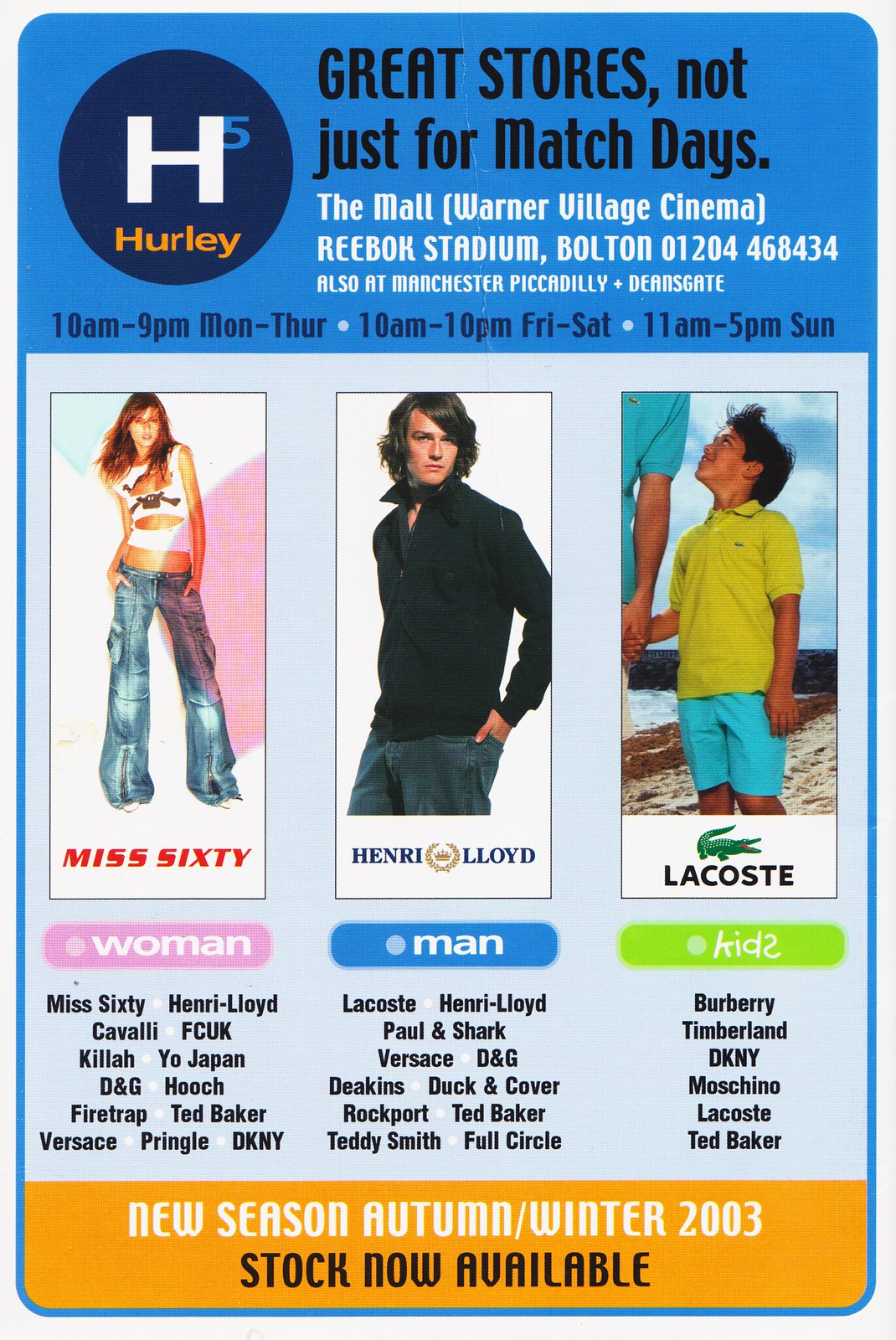This is an advertisement featuring vibrant hues of blue, white, and yellow, with additional accents in pink, green, light blue, tan, and black. Set against a blue backdrop, the top of the ad prominently showcases the slogan "Great Stores, Not Just for Match Days" in black text. Below, the advertisement details locations: "The Mall, Warner Village Cinema, Reebok Stadium, Bolton, 01204-468-434, also at Manchester Piccadilly and Dean's Gate." To the left, a dark blue circle with a prominent white "H" and the number "5" in blue, highlights "Hurley" in yellow text. The operation hours are listed beneath in dark blue: "10 a.m. to 9 p.m., Mon to Thur, 10 a.m. to 10 p.m., Friday, Saturday, and 11 a.m. to 5 p.m., Sunday."

Central to the ad are three professionally shot images, set against a white background. The left image shows a brunette woman in a white crop top and denim, labeled "Miss 60" in red. The middle image features a man with shoulder-length brown hair, wearing a black zip-up shirt and dark denim, labeled "Henry Lloyd." The right image depicts a child with dark hair in a yellow polo and teal blue shorts, standing on a beach, labeled "Lacoste."

Under each image, corresponding tags categorize the models: "Woman" in a pink circle beneath Miss 60, "Man" in a blue circle beneath Henry Lloyd, and "Kids" in a green circle beneath Lacoste. Below these tags, brand names are listed under each category. For "Woman" and Miss 60: Cavelli, FCUK, Killa, Yo Japan, D&G, Hooch, Firetrap, Ted Baker, Versace, Pringle, and DKNY. For "Man" and Henry Lloyd: Lacoste, Henry Lloyd, Paul and Shark, Versace, D&G, Deacons, Duck and Cover, Rockport, Ted Baker, Teddy Smith, and Full Circle. Under "Kids" and Lacoste: Burberry, Timberland, DKNY, Moschino, Lacoste, and Ted Baker.

At the bottom, the ad features a yellow-gold background with the announcement "New Season, Autumn/Winter 2003" in white letters and "Stock Now Available" in black letters.